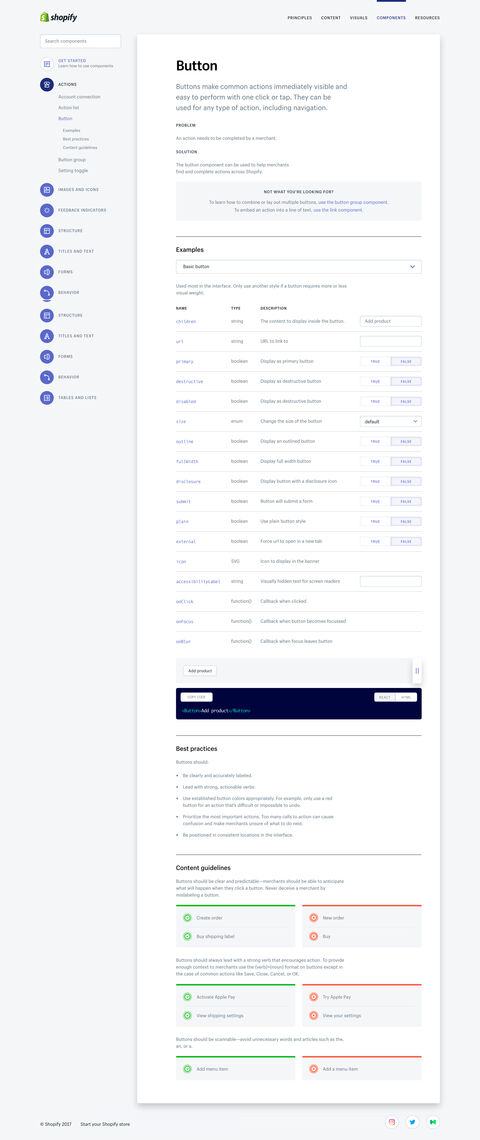This is a detailed screenshot of a Shopify interface. The recognizable Shopify logo, a green shopping bag with an "S" on it, is positioned at the top left corner. Just below the logo, there is a search bar. Beneath the search bar, there are two prominent tags: one labeled "Get Started" and another marked "Actions." Below these tags, there are more than ten icons arranged vertically.

Occupying the majority of the page on the right is a section with a white background. The top of this section displays a button, positioned above a chart titled "Examples." This chart features a dropdown menu, which, despite zooming in, remains difficult to read clearly. The far right column of this chart contains boxes marked "True" and "False," with the "False" boxes shaded a lighter gray compared to the "True" boxes.

At the bottom of the page, there's another chart with a blue header labeled "Best Practices." Listed under this header are approximately four or five bullet points. The final section of the page is titled "Content Guidelines." This section showcases color-coded boxes: on the left side, there are three boxes with only their top lines colored green, and on the right side, there are three boxes with top lines colored orange.

Overall, the page is organized into sections that include action tags, a detailed chart with examples, best practices, and content guidelines, providing a comprehensive view of the Shopify interface.